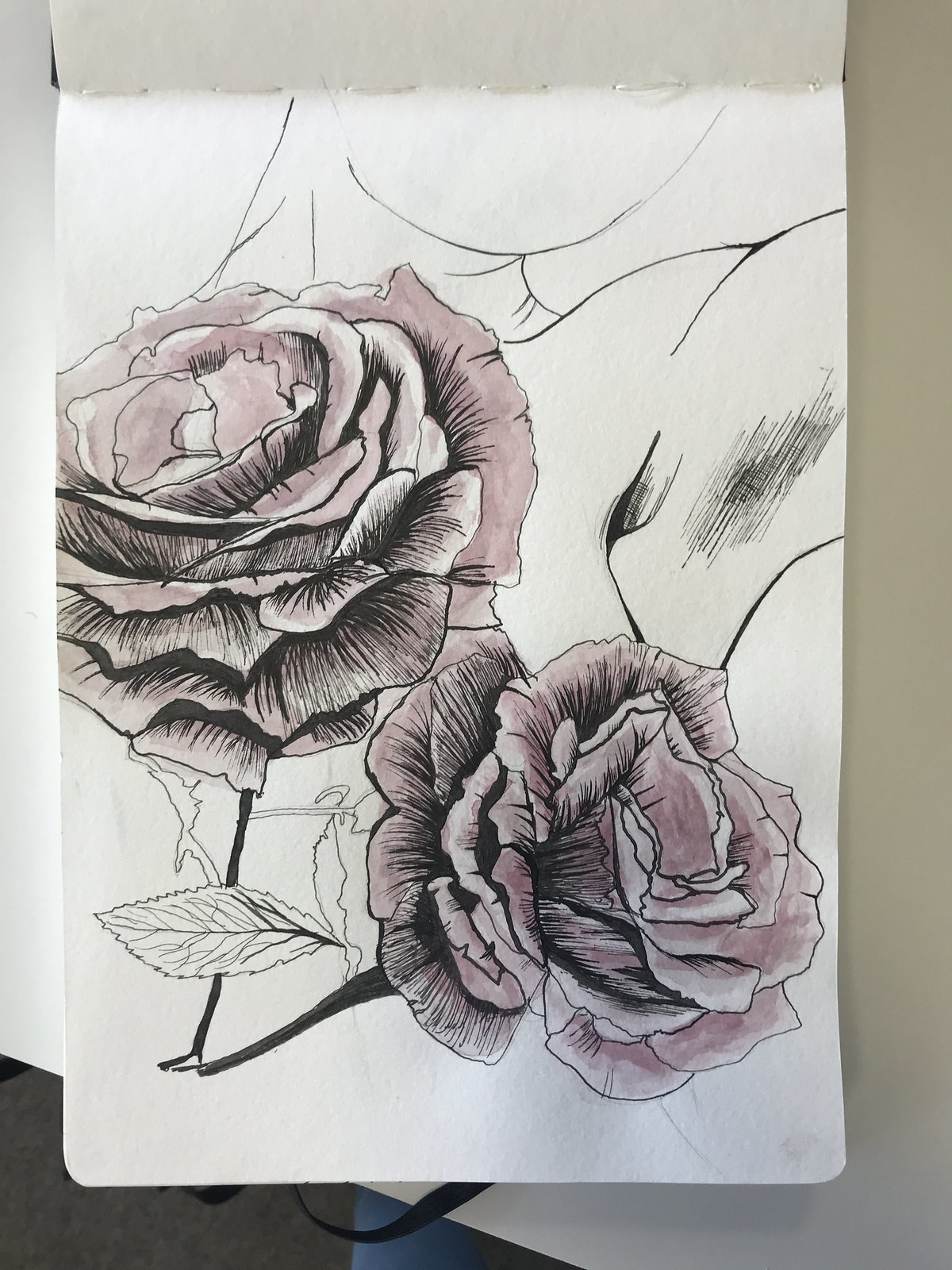A vertically oriented image captures an open sketchbook placed on a white table. The visible page showcases an intricate black pen drawing of two roses laid across a person's chest. The roses are partially colored with a muted mauve marker, adding a delicate touch of pink. The shading is expertly done with the black pen, creating depth and dimension. In the background, the lower part of the person's face, including their chin and neck, is visible, along with one of their underarms. The roses dominate the composition, drawing the viewer's attention to their detailed and artistic rendering.